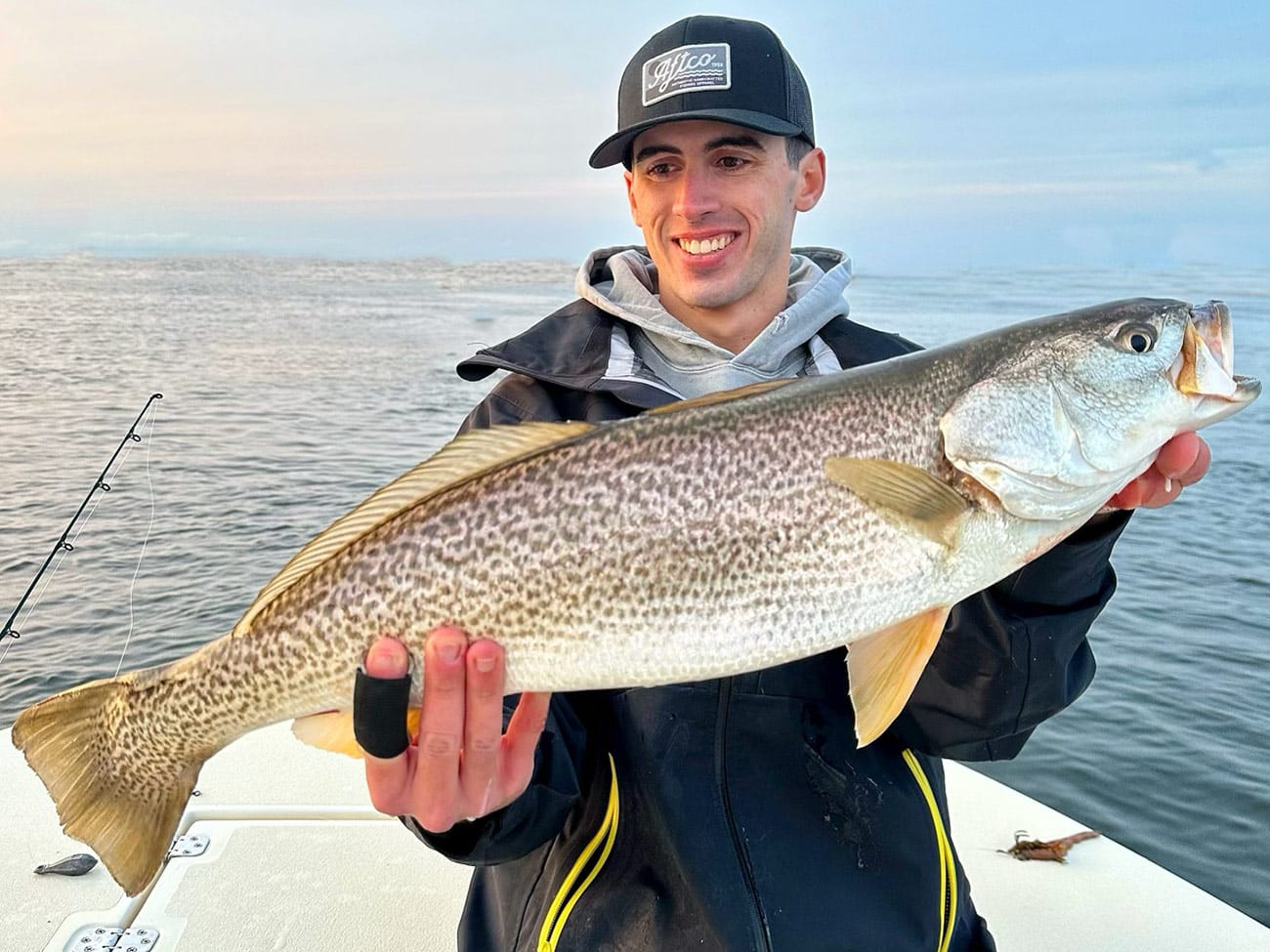In this photograph, a man is prominently showcased holding a large, grey-yellowish fish with dark spots and an open mouth. Captured from the hips upward, he stands on a white boat with a clear, light blue sky and a calm, darkish ocean in the background, likely in the early morning or near dusk given the soft lighting. The man is smiling widely, looking towards his right and slightly down at the fish. He is dressed in a blue baseball cap with "Aftco" lettering, a gray sweatshirt with a hood, and over that, a dark blue or black parka featuring yellow detailing on the pockets. Notably, he also has a black bandage wrapped around his right forefinger. Visible in the background is part of a fishing rod, reinforcing the notion that he has just caught the fish. The serene scene is indicative of a peaceful moment on the water.